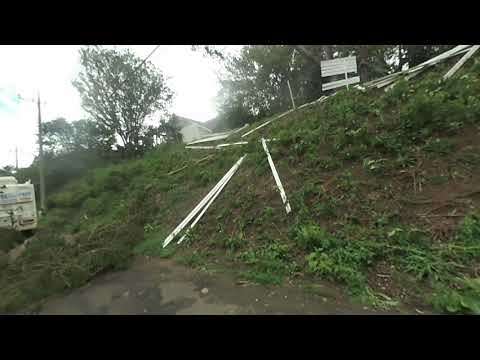In this landscape-oriented color photograph, a hillside is depicted post-storm. The sky appears hazy and very white, creating a stark contrast with the scene below. The hillside, covered in patches of dirt and green grass, ascends from the left to the right. At the hill's bottom, muddy, brown floodwater reflects light.

In the left-hand corner, the sparse branches of a tree on the slope are visible with more trees ascending the hill. Behind this tree, partially hidden, is a white RV parked under a lamppost. White sticks or pieces of wood—debris from a disassembled sign—are scattered across the hillside. These pieces are seen strewn from the sign at the top right of the image to the center, indicating the storm's impact. 

Additionally, a house peeks through from the top left of the hillside, adding to the setting's realism. The style of the photograph is representationalism realism, capturing the detailed and chaotic aftermath of a storm in a rural landscape setting.